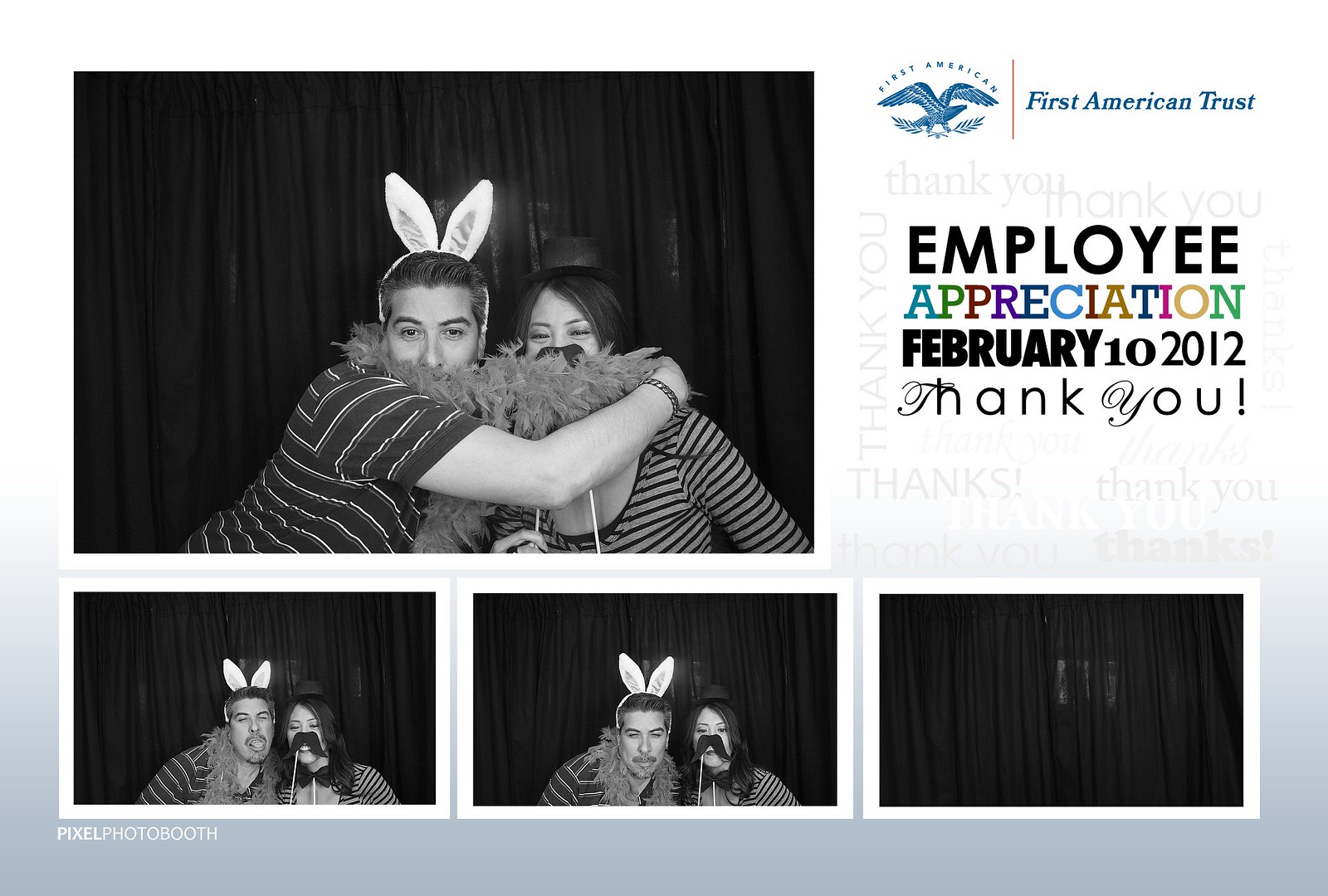The image is a collage of photos set against a black and white backdrop, capturing a playful moment from an employee appreciation event. In the top right corner, a blue logo featuring a bird is displayed alongside the text "First American Trust" on a white background. Below this, the text reads "Employee Appreciation, February 10, 2012" followed by a "Thank you" in a different font. The main section on the left features a large black and white photo of a man and woman dressed up with props: the man sports rabbit ears and a feather boa, while the woman wears a striped shirt and holds a mustache on a stick with a top hat nearby. They stand in front of a dark curtain. Below this main photo are three smaller black and white images arranged horizontally: the first two capture the pair making funny faces, while the third shows an empty black curtain. The bottom left corner of the collage reads "Pixel Photo Booth."